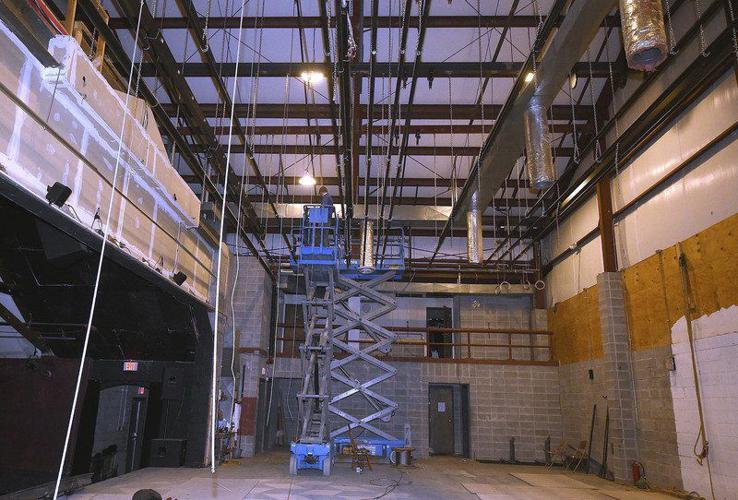The image captures an expansive warehouse construction site, characterized by its brick and stone walls. To the left, an open area with an illuminated exit sign above an open doorway connects to an area of visible drywall undergoing work. Above this section, the open ceiling reveals a grid of beams crisscrossing both horizontally and vertically, indicating an unfinished roof with exposed rafters. The warehouse floor is unfinished, covered with plywood, and hosts two pieces of heavy machinery designed for lifting workers to higher levels. In one lift, a Caucasian man is visible operating the equipment. The setting is well-lit, showcasing various shades of brown from the plywood and rafters and gray from the stone and brick walls. The overall scene is vibrant with construction activity, emphasized by hanging ropes from the ceiling and detailed structural elements that suggest ongoing remodeling efforts.